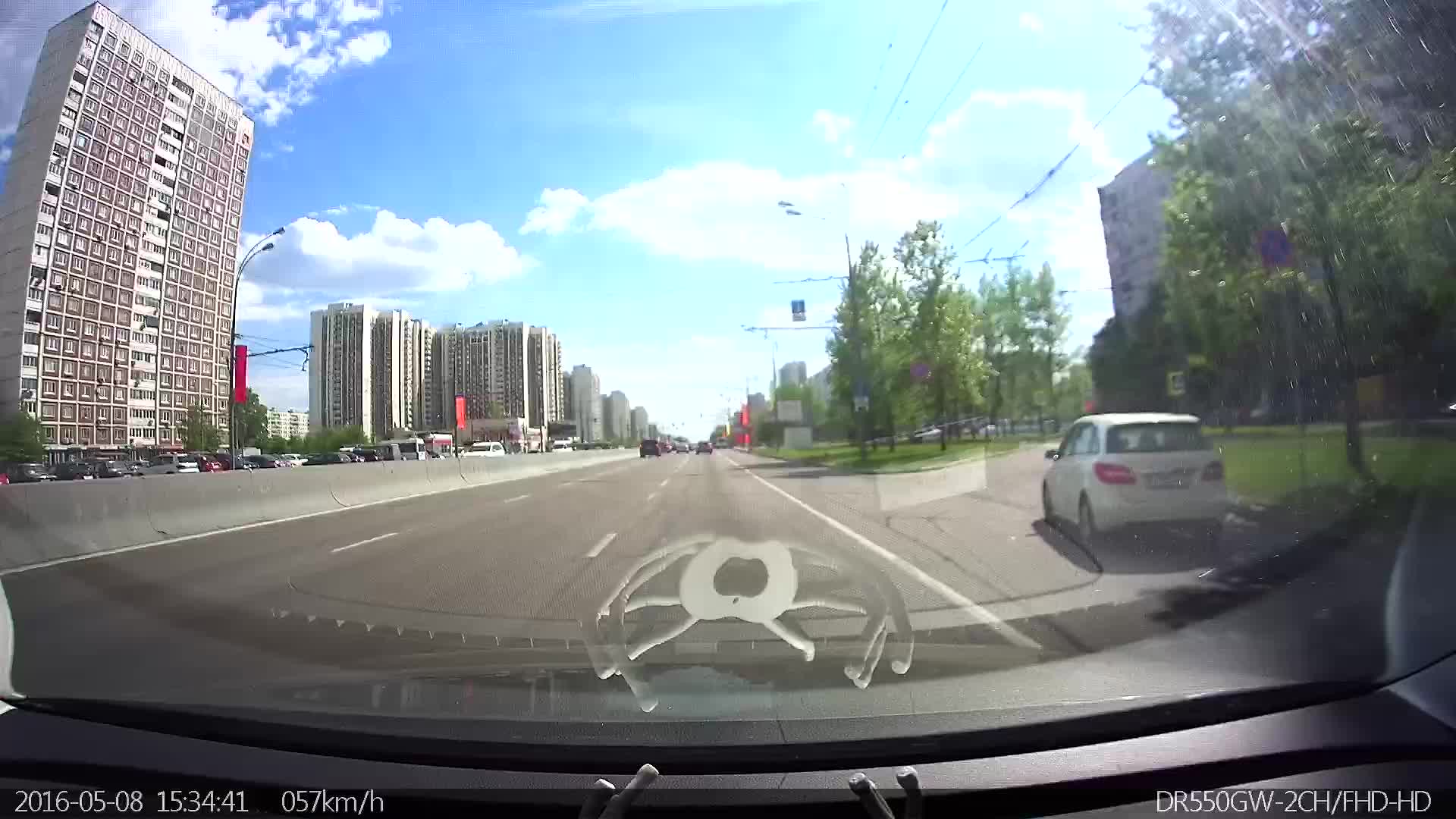This image appears to be a highly detailed 3D rendering mimicking a dash cam view. The 3D artistry is evident due to the overly uniform buildings on the left, which feature identical window designs and lack depth, resembling a fish-eye effect. At the bottom of the image, there are various speed measurements displayed, such as 12, 16, 5, 8, 15, 34, 41, and 57 kilometers per hour, along with the specific model of the dash cam. The car dashboard and windshield are visible at the bottom edge of the frame. On the right side, a car is seen turning into what appears to be a valet parking area next to a building, surrounded by numerous trees. The scene is set on a wide six-lane road, with three lanes in each direction, under an overcast yet bright blue sky.